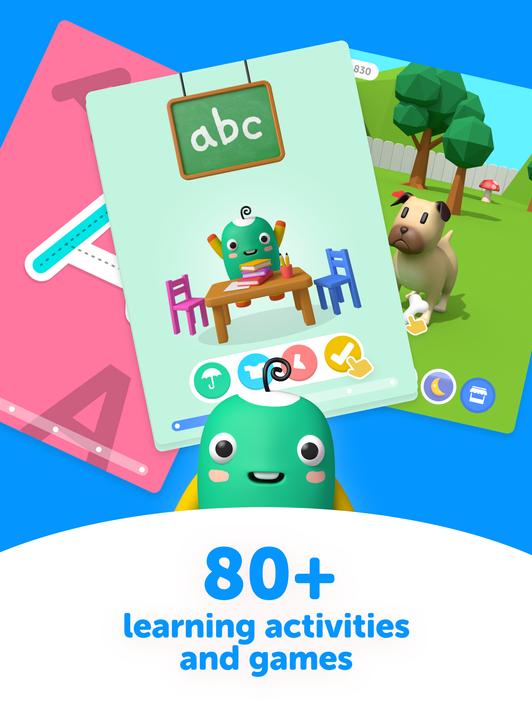Sure, here's a cleaned-up and detailed caption for the image based on your description:

---

Screenshot of a vibrant and playful virtual advertisement against a blue backdrop. At the top, the ad features the phrase "80+ Learning Activities and Games" in white text. The advertisement is divided into three sections with distinct images. 

The first section showcases a charming green creature seated beside a desk with two adjacent chairs—one blue and one purple. The desk displays icons representing a green umbrella, a blue shirt, a red bird, and a yellow check mark, with one icon selected. An ABC board is mounted just above the desk, enhancing the educational theme.

The second section of the advertisement presents an illustration of a dog amidst green trees, evoking a sense of outdoor adventure and learning.

The third section, set against a purple background, includes another creature at the bottom, although details are less distinct in this part of the image.

The overall design emphasizes a fun, engaging educational experience for children with a variety of learning activities and games.

---